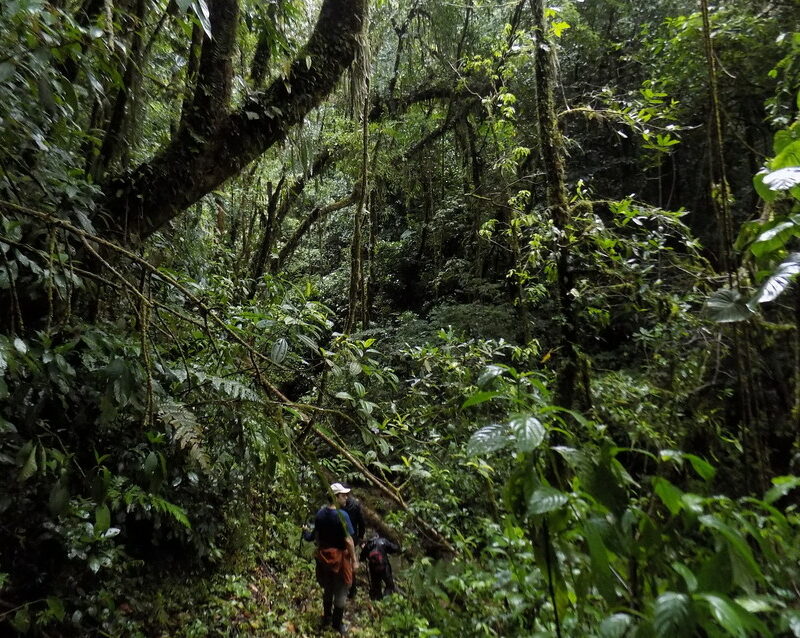This image captures a scene deep within a dense tropical rainforest, where the lush greenery and thick vegetation create an almost impenetrable backdrop of vines, moss-covered branches, and towering trees. Daylight struggles to penetrate the dense canopy, casting a dim, verdant glow over the forest floor. In the foreground, two hikers traverse a narrow trail; one, slightly ahead, sports a red backpack. The second hiker wears a white baseball cap, a blue cotton t-shirt, grey pants, black boots, and an orange jacket tied around his waist. The overwhelmingly verdant surroundings dwarf the hikers, emphasizing the vast, untamed nature of the jungle.